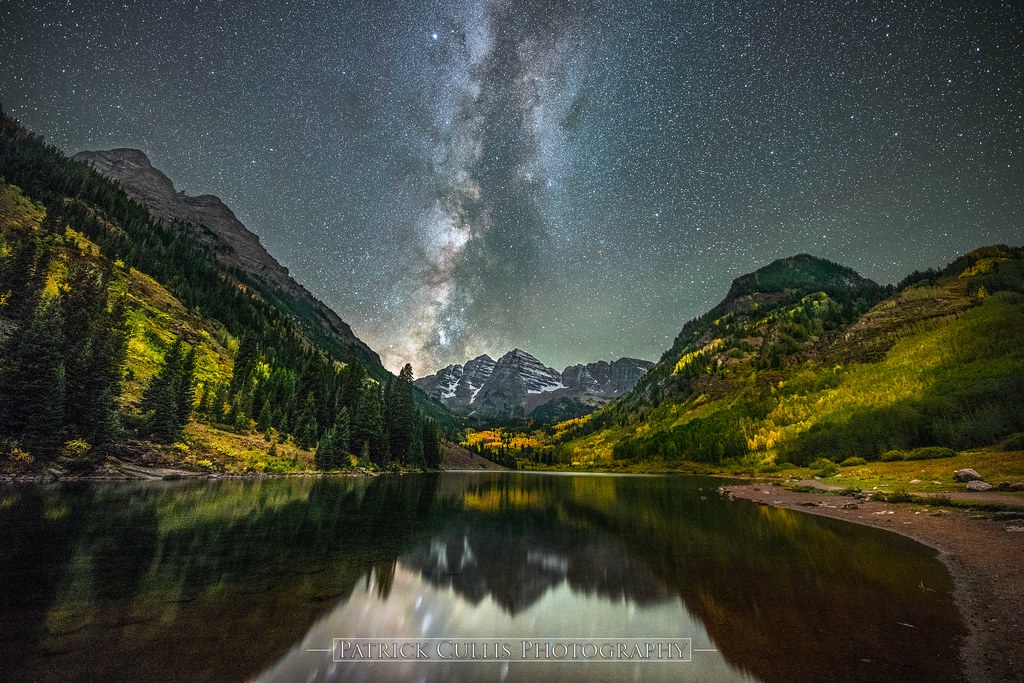This detailed painting depicts a serene lake flanked by towering mountains on either side. The mountains closer to the viewer are lush with greenery, extending upwards with grass and densely packed trees. The mountain to the left features a rugged, rocky summit. Further in the distance, the majestic high-peaked mountains are capped with glistening snow. The scene is set under a night sky studded with stars, where faint moonlight filters through scattered clouds, casting a gentle glow across the heavens. The tranquil water of the lake mirrors the surrounding mountains and the partially obscured, luminous night sky, creating a stunning reflection in the dark, shimmering surface.